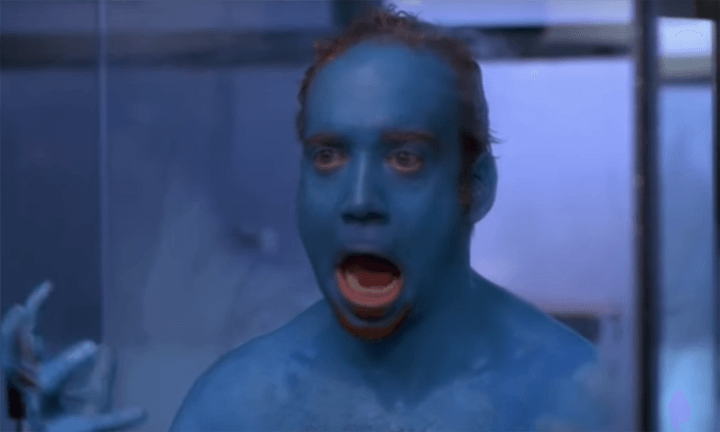This image is a vivid portrayal of a man who is completely painted in a bright, vibrant blue, reminiscent of the Blue Man Group. His entire body—from his face, chest, neck, and ears to his hands and fingers—is covered in blue paint. He stands shirtless, revealing his painted torso. His mouth is agape, showcasing pink and red accents inside his mouth, with visible teeth and tongue, and his eyes are wide open, giving the impression that he is screaming or yelling at himself in the mirror. The man has distinct black hair and a black beard, contrasting starkly with the blue paint on his skin. The background, slightly blurred and tinged in blue and white light, suggests he might be in a bathroom. There appears to be a black windowpane visible in the backdrop. The overall scene could be a humorous movie screenshot, potentially involving actor Paul Giovanni, who is caught in a moment of shock and disbelief as he stares at his own reflection, seemingly bewildered by his entirely blue appearance.